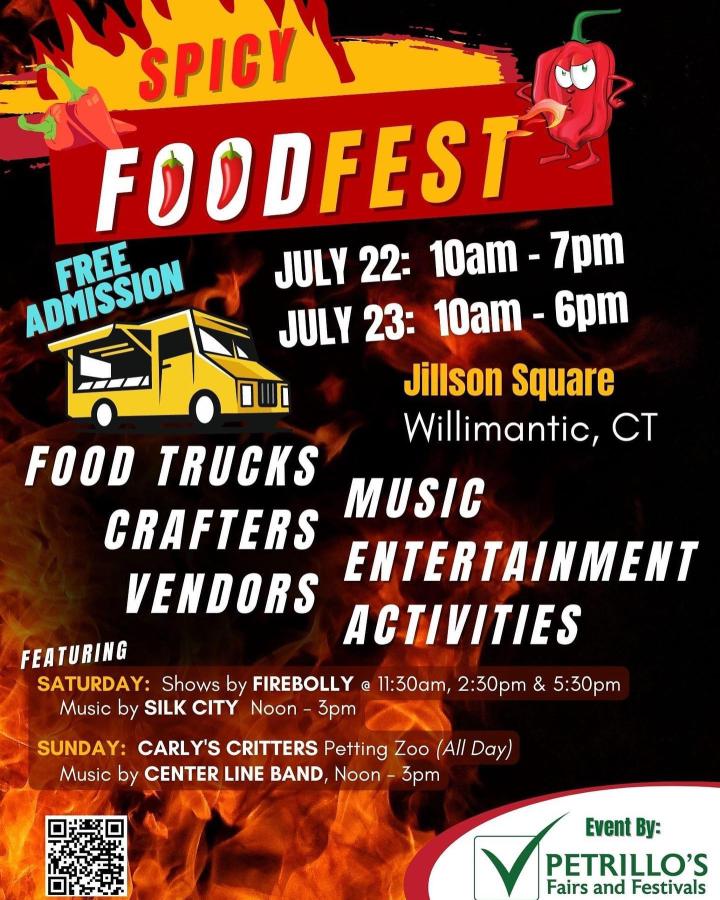This vibrant and eye-catching brochure advertises a "Spicy Food Fest" event, prominently featuring a fiery theme. The top of the brochure showcases bold red text that says "Spicy" with flaming accents and an artist's rendition of fire shooting up. Adjacent to this are the words "Food Fest" displayed in a red textbox, with "Food" in white and "Fest" in yellow. The O's in "Food" are cleverly replaced with chili peppers. 

A cartoon bell pepper with green eyes and flames spewing from its mouth stands to the right, striking a confident pose with hands on hips. Below this are the event details: July 22nd from 10 AM to 7 PM and July 23rd from 10 AM to 6 PM, taking place at Gilson Square in Willimantic, Connecticut. 

To the left of these details is an image of a food truck with its serving window open, and above it in cyan text, it reads "Free Admission." Underneath the dates and location, a white text list highlights the event’s offerings: food trucks, crafters, vendors, music, entertainment, and activities.

Near the bottom, the schedule specifies featured activities: Saturday shows by Fire Bully from 11:00 AM to 2:30 PM and 5:30 PM, and music by Silk City from noon to 3 PM. Sunday includes Carly's Critters Petting Zoo all day, and music by Centerline Band. 

The bottom corners contain additional information: a QR code on the lower left, and in the lower right, a white oval with green lettering announcing "Event by Petrillo's Fairs and Festivals." The entire design features shades of red, yellow, and black, reinforcing the spicy and fiery theme of the event.